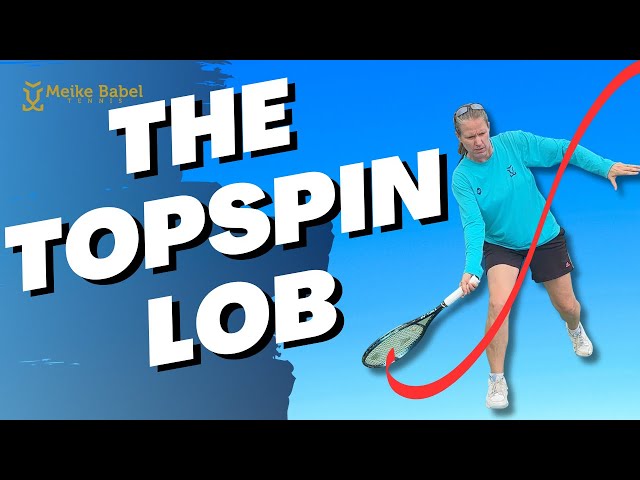The thumbnail image for the video titled "The Top Spin Lob" prominently features a tennis player in action, swinging a racket with a dynamic red arrow illustrating the motion. The player, who has pale skin and short hair, is dressed in a teal blue long sleeve shirt, black shorts, white socks, and white tennis shoes, with goggles resting on top of their head. The background features a two-tone blue gradient, darker on the left and lighter on the right, with black bars at the top and bottom of the image. The text “Mieke Babbel Tennis” is displayed in small gold letters in the upper left corner, and the title "The Top Spin Lob" is prominently seen in large white letters. The overall composition vividly captures the instructional focus on the tennis technique being highlighted.